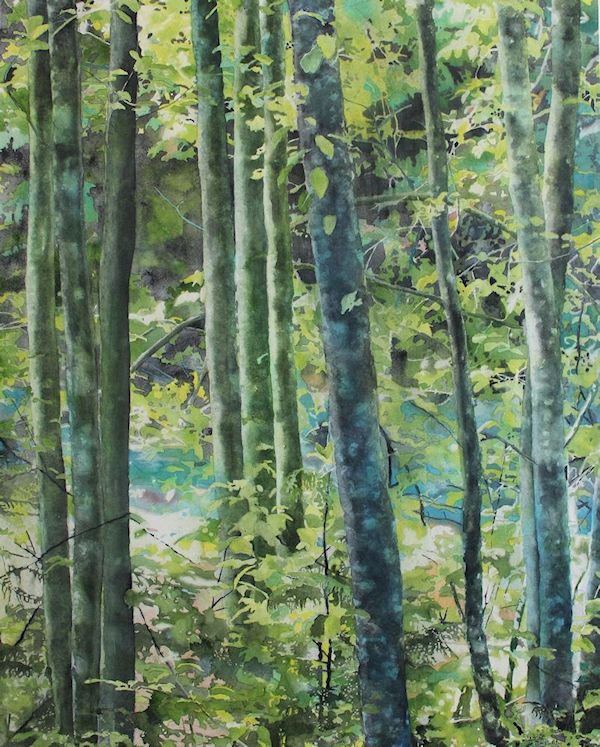The image is a rectangular painting of a forest scene, capturing an outdoors setting with numerous tall, thin tree trunks adorned with soft, blurry green leaves. The trunks, notable for their splotchy blue-gray color, appear in clusters—three bunches situated towards the left, one bunch in the center, and several trunks along the right side. At the forefront, a lone tree stands out with markings suggestive of mold, algae, moss, or fungus. The painting's palette is composed of subtle colors, including green, blue, pink, and white. Amidst the dense assembly of branches and twigs, there seems to be a watery lake partially obscured by lush greenery, hinting at the scene's depth. The overall image, though crowded with foliage and tree trunks, provides a straightforward depiction of a wooded area.